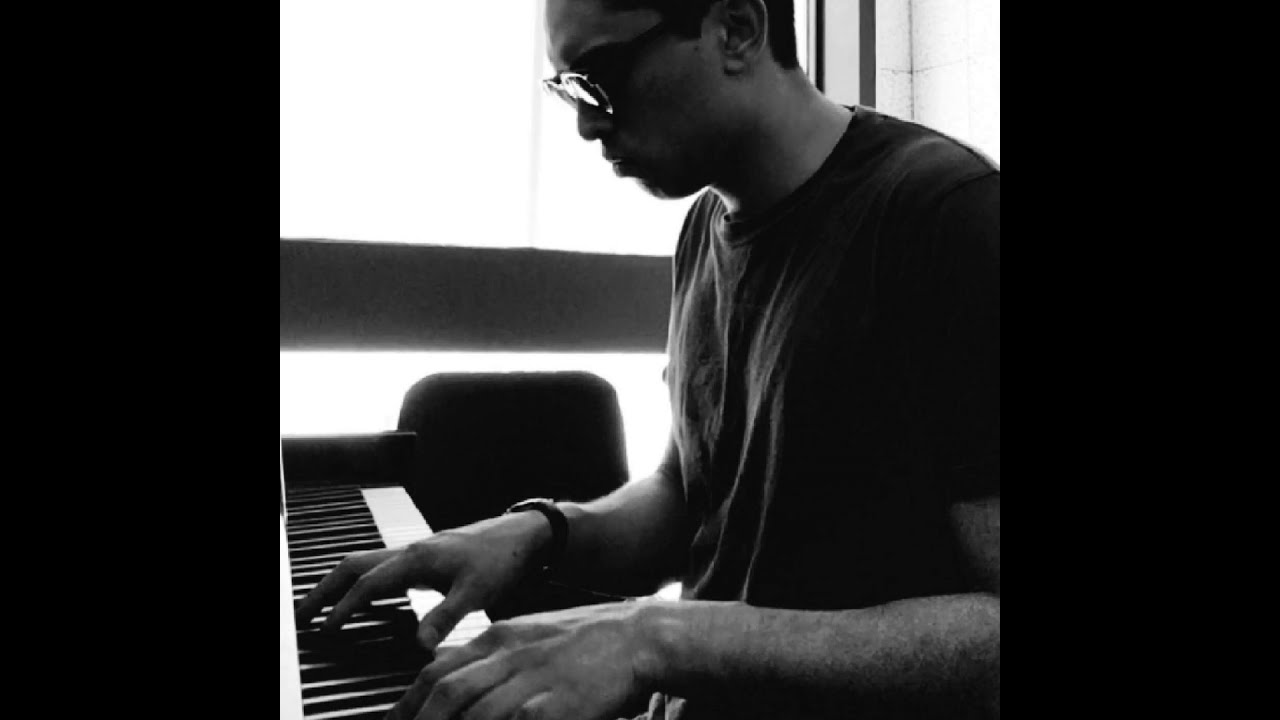This is a detailed black and white photograph of an Asian man playing the piano, styled like a social media post. The image, rectangular and horizontally oriented with vertical black stripes on either side, centers on the man who is slightly off to the right. He is intently looking to the left, possibly at sheet music. He wears glasses, a dark short-sleeved t-shirt, and a watch on his left wrist. His dark hair and serious expression suggest a focused moment. His fingers rest on the keys of the piano at the bottom left of the image. The top half of the background features an overexposed window, indicating it is daytime. A light stripe runs horizontally across the window, bisecting the overexposed light. Below this, a chair and light-colored walls are visible, situating the scene in a music room. The overall composition highlights the contrast between the detailed, engaged subject and the stark, bright background.